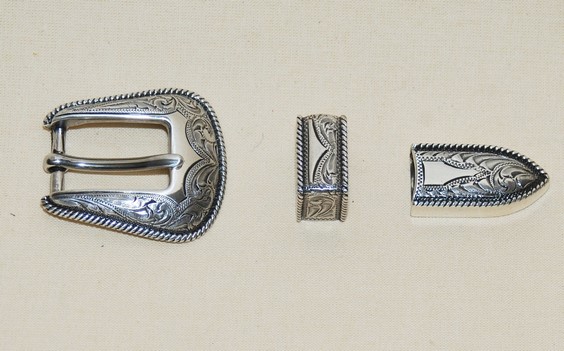The image shows three detached, shiny metal parts of a belt, laid out horizontally on a white or slightly off-white surface. The objects appear to be made of stainless steel or a similar silver-toned metal, possibly pewter, with intricate black engravings on their edges. On the left is an ornate belt buckle adorned with swirling wave-like patterns and an elegant rectangular centerpiece. The buckle’s latch part faces left. The middle piece is the belt loop, featuring matching ornate designs intended to secure the belt's end. The rightmost piece, resembling a pointed tail, fits on the belt's tapered end, echoing the design motifs of the other parts. Each piece showcases ridges along the edges where the black engravings are embedded, enhancing the overall decorative appeal. The image is likely intended for a product listing, showcasing this ornamental belt hardware in a clear, detailed presentation.